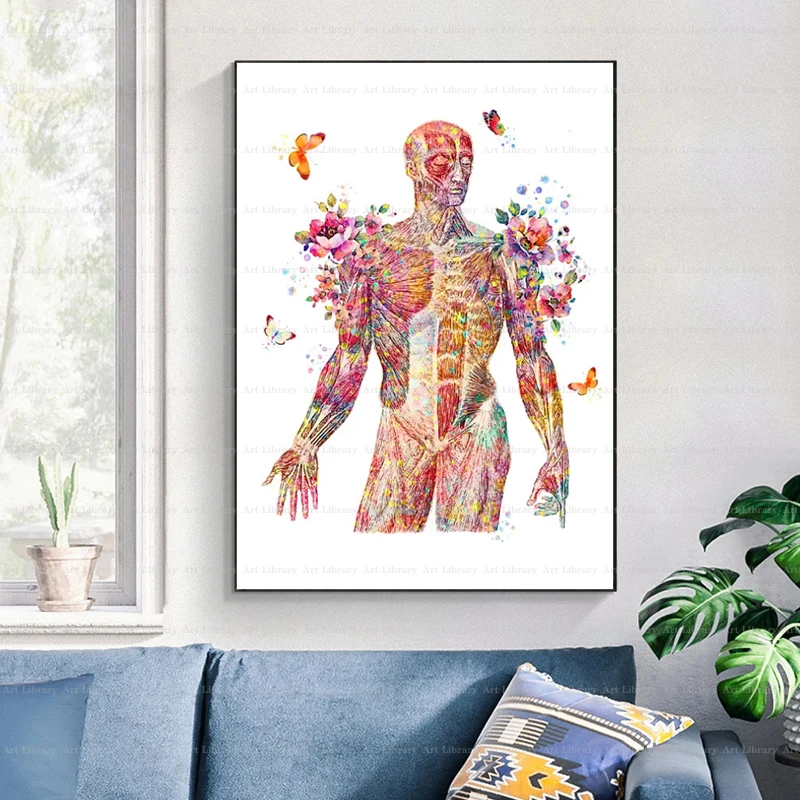The image captures a detailed depiction of a living room, with the main focus being a striking painting above a blue couch. The painting showcases a human body devoid of skin, intricately revealing the muscle groups in a vibrant rainbow of colors. The shoulders of the figure are adorned with colorful flowers bursting forward, and pollen seems to scatter around them. Four butterflies—an orange one, a reddish one, a whitish one with purple wingtips, and another unmentioned—are fluttering around the flowers. The artwork is encased in a thin black frame, making the vivid colors stand out against its white background.

To the left of the painting is a window with a gray and white frame, through which faded trees can be seen outside. On the windowsill rests a brownish-colored potted plant with lush green leaves. Below the painting is a blue couch, accentuated by a yellow-and-blue pillow with striped patterns. On the right side of the image sits another larger potted plant in a silver pot, sporting big green leaves. The entire scene is set against a clean, white wall, contributing to an overall sense of brightness and tranquility in the room.